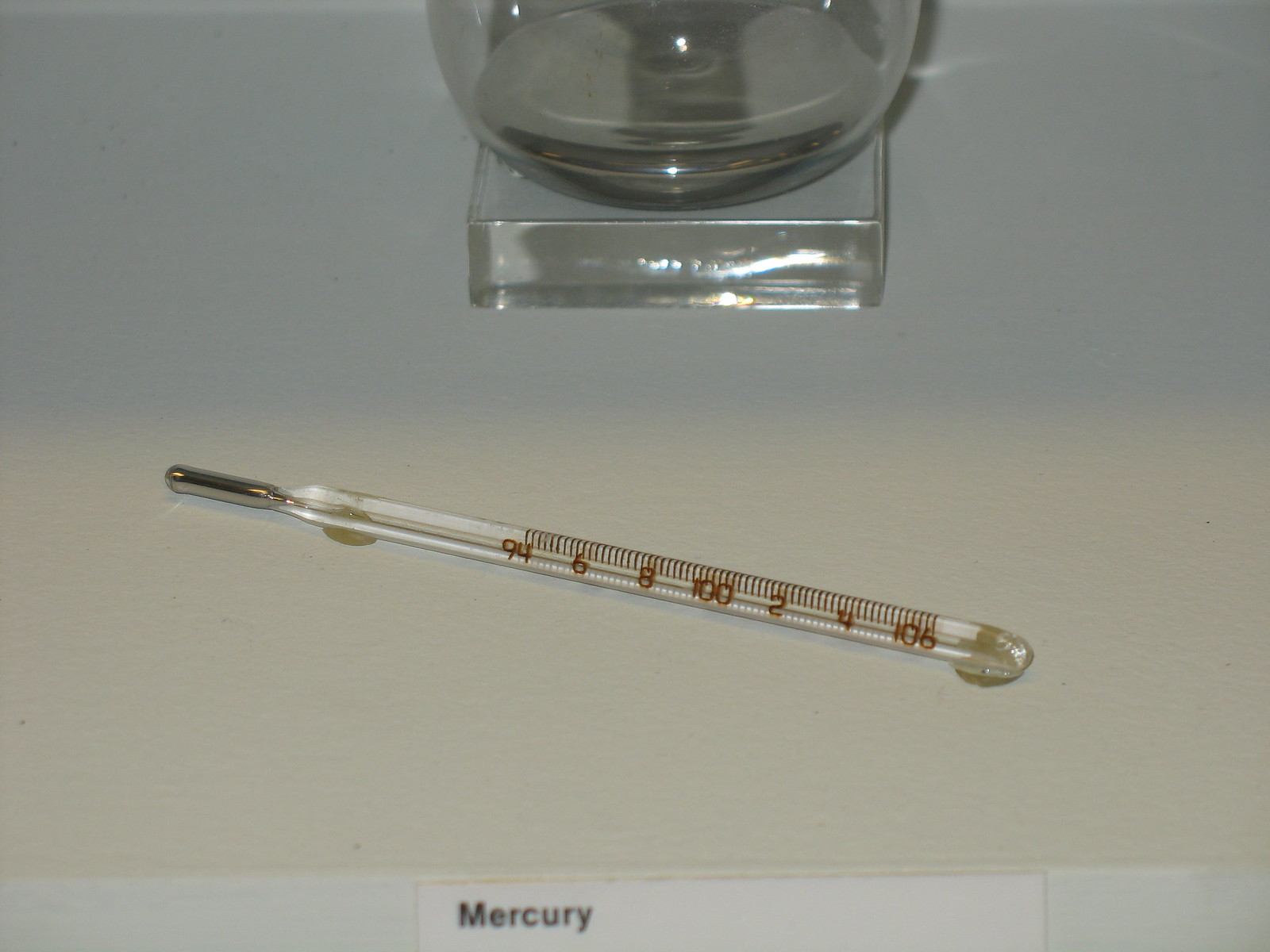The image captures a vintage glass mercury thermometer, reminiscent of those used several decades ago. The slender, oblong thermometer features a shiny silver tip designed to be placed under the tongue. The glass body is marked with a temperature scale ranging from 94 to 106 degrees Fahrenheit, with numerous small notches indicating possible readings within that range. The thermometer is resting on a pristine white table, and currently, it does not display any specific temperature reading. Positioned above the thermometer is an enigmatic glass object with a clear square base and a rounded top, likely a decorative piece, although it is partially cropped out of the image. Imprinted at the bottom of the photo in black lettering is the word "mercury," highlighting the thermometer's old-fashioned design which employs the now largely discontinued substance.